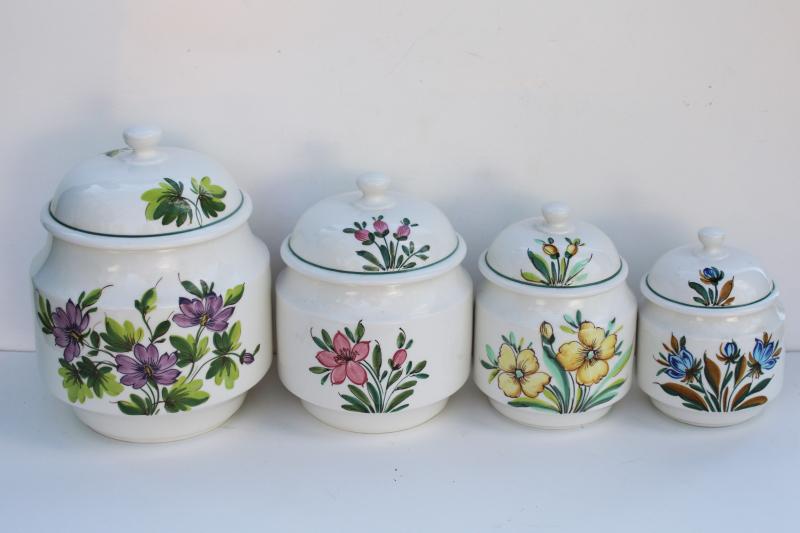This photograph features a set of four white ceramic containers, each elaborately decorated with hand-painted floral patterns. Arranged from left to right in ascending order by size, each container progressively increases in height. The smallest container, positioned on the right, is adorned with delicate blue flowers accompanied by brown stalks and green leaves. Moving leftward, the next container displays yellow blossoms amidst green foliage. The third container features vibrant magenta flowers with green leaves. The largest container on the far left boasts an array of purple flowers with lush green leaves. All four containers sit on a white countertop against a similarly white backdrop, with a faint shadow and the subtle presence of a light source, possibly from the flash used to take the picture, casting soft highlights in the background.